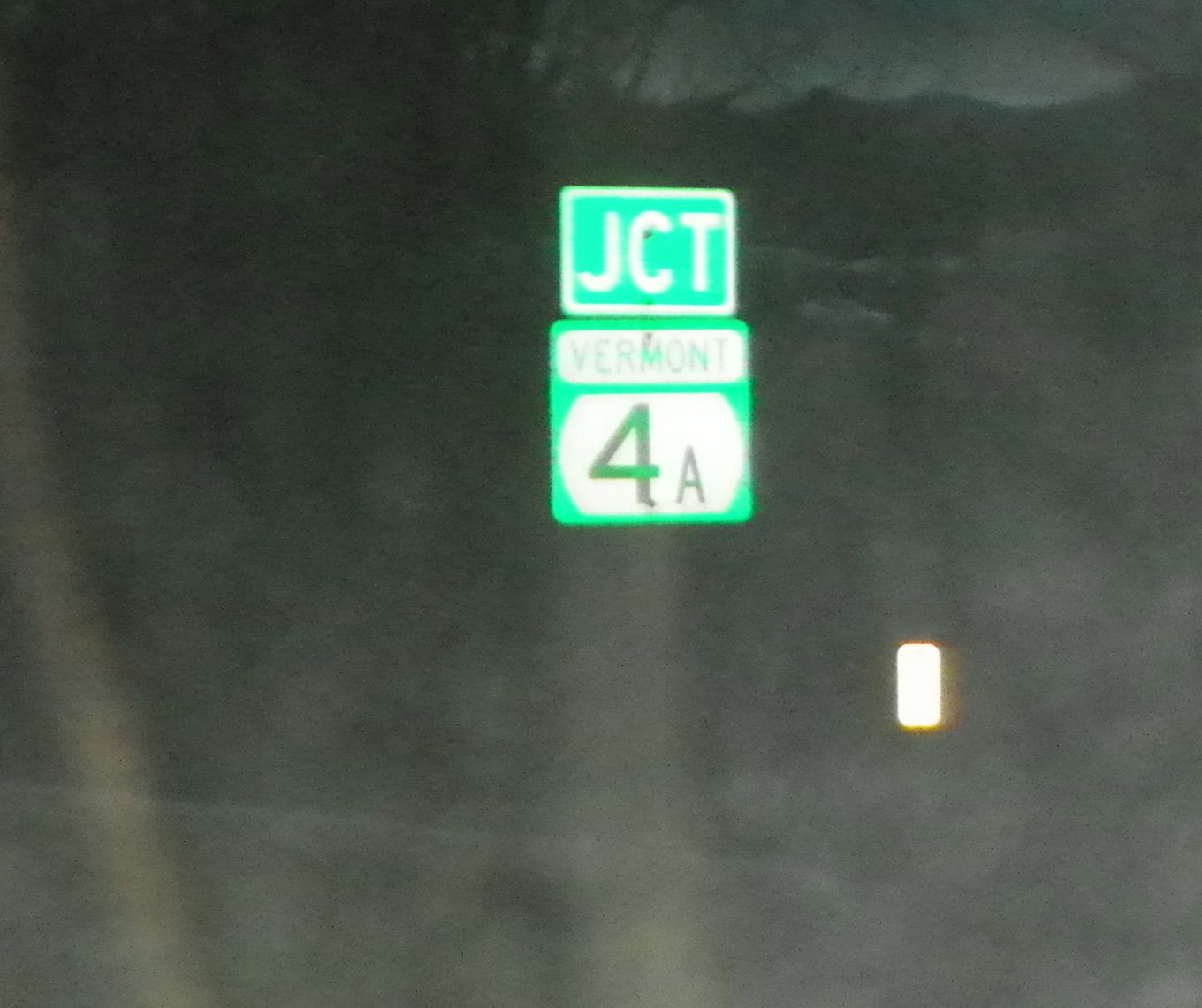A nighttime photograph depicts a street sign intersection in Vermont. The image focuses on two signs affixed to a pole: a smaller rectangular sign at the top reading "JCT" (junction), and a larger square sign beneath it indicating "Vermont 4A." Despite the pervasive darkness, the pole is faintly visible. The upper portion of the photo features silhouettes of tree branches against a dimly lit sky, adding to the moody atmosphere. On the right-hand side, approximately two-thirds down from the top, a vertical rectangular patch of light appears, possibly a reflection, subtly illuminating that portion of the image.